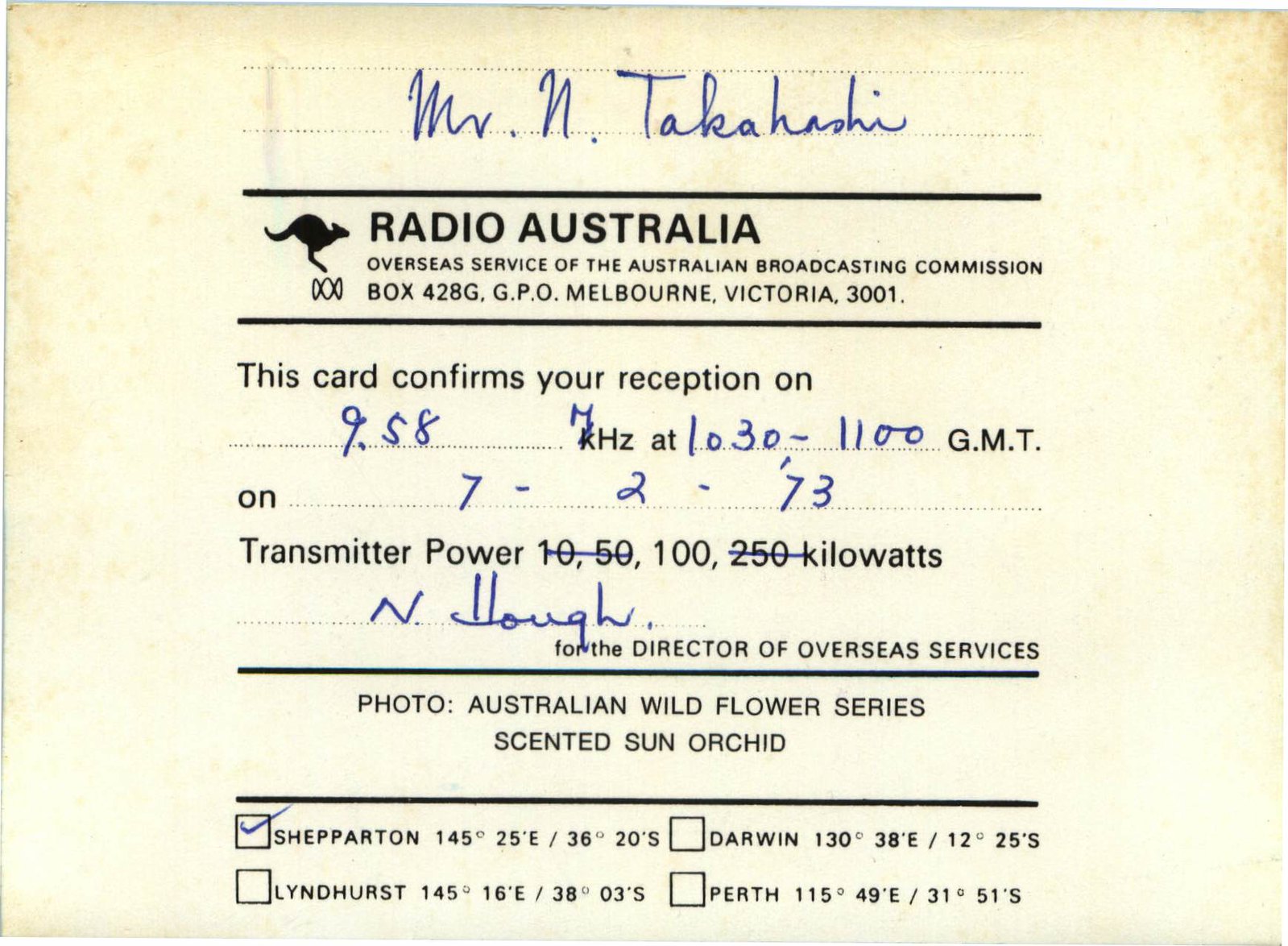The image depicts an aged, yellowish-grey piece of paper, which appears to be correspondence from the Radio Australia Overseas Service of the Australian Broadcasting Commission. The top of the document features a blue handwritten note addressing Mr. N. Takahashi, followed by a thick black line. Below the line is a logo of a kangaroo, and next to the logo is the typed text "Radio Australia, Overseas Service of the Australian Broadcasting Commission, Box 428G, GPO Melbourne, Victoria 3001." Another thick black line follows beneath this text. 

The main body of the document confirms the reception of a broadcast, with the typed message: "This card confirms your reception on 9587 kilohertz at 1030 to 1100 GMT on 7-2-73. Transmitter power: 100 kilowatts." Notably, the numbers 10, 50, and 250 kilowatts have been crossed out by hand in blue ink. The message is signed "N. Hugh" for the Director of Overseas Services. 

Below this, the document mentions "Photo Australian Wildflower Series: Scented Sun Orchid," yet no such photo is present. At the bottom, there are four checkmark boxes—one each for Shepparton, Lyndhurst, Darwin, and Perth. Only the box for Shepparton is checked, with coordinates "145 degrees 25' east, 36 degrees 20' south" annotated beside it. The card conveys a blend of typed precision and personal handwritten touches, denoting a formal yet personalized piece of communication.